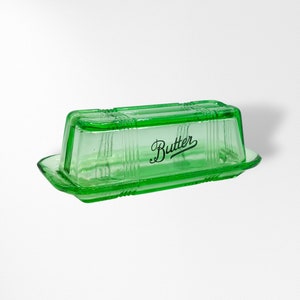This square photograph, taken indoors against a light gray backdrop that merges with the ground, showcases a distinctive butter holder. The holder is crafted from translucent glass or possibly acrylic, tinted with a green hue. Central to the image, the butter dish appears to be suspended and casts a shadow on its right side, indicating a light source from the left. The dish comprises a tray-like base with a removable top, both tinted green. Prominently displayed on the side of the top piece, the word "butter" is elegantly inscribed in black cursive, starting with a capital B and ending with the R extending into an underline beneath the word. The overall effect blends the green-tinted translucence with the simplicity of the gray background, emphasizing the butter dish's unique design.